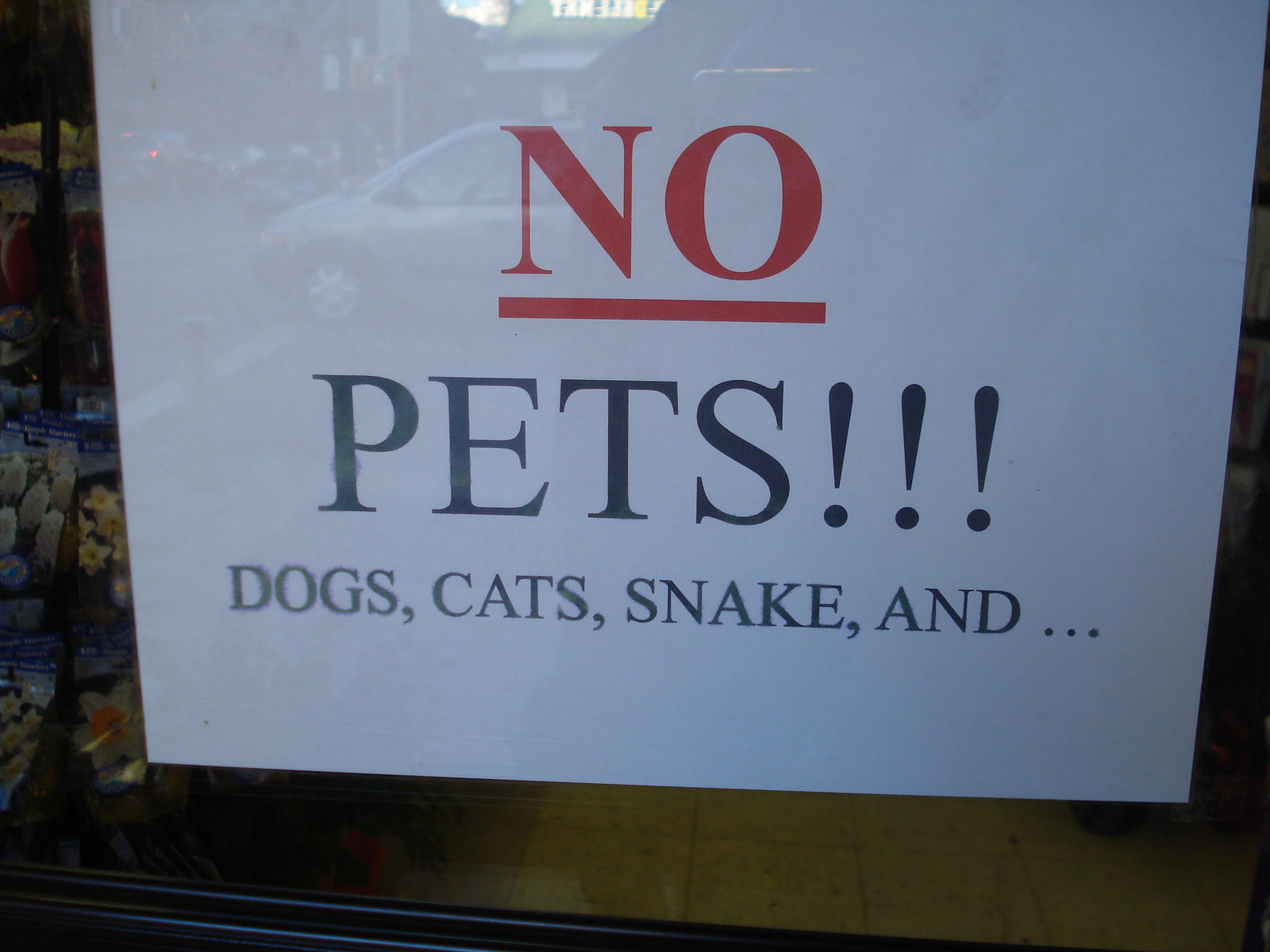The image depicts a prominently displayed sign taped to the inside of a store window, clearly intended to communicate a strict no-pets policy. The sign dominates the image with its large, bold capital letters, making the message unmissable. At the top of the sign, the word "NO" is written in red, underlined for emphasis, followed by "PETS!!!" in black, equally bold text. Beneath this, a smaller-font line lists specific animals - "Dogs, Cats, Snakes," followed by an ellipsis, underscoring an all-encompassing prohibition on pets.

The sign is fixed behind a glass pane, through which various reflections reveal a street scene with several vehicles, including a minivan. The store's interior is partially visible, showing a light-colored tile or linoleum floor and a silver rim at the window's bottom edge. There are flowers or possibly bouquet packets visible on the left side of the image, hinting at the store's business.

The reflections and the detailed list of prohibited animals suggest that the store has had repeated issues with customers attempting to bring in their pets, prompting this definitive notice.